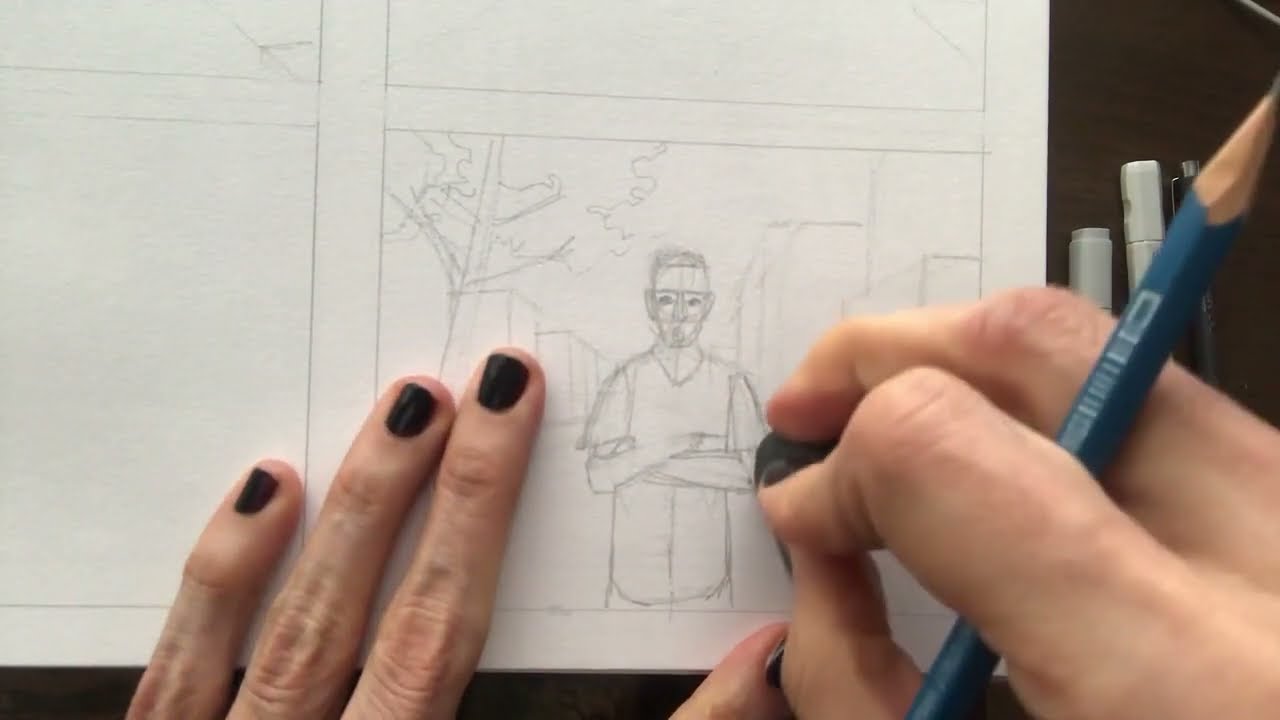The image depicts a detailed close-up scene of an artist at work, captured in a horizontally aligned rectangular picture. Two slender hands with light-colored skin and black nail polish are visible at the bottom of the image, engaged in the process of sketching. The right hand, holding a blue wooden pencil, is actively drawing on a piece of white paper. The paper is sectioned into four squares, with the bottom right square prominently displayed. In that square, the artist is drawing the front view of a man with short hair and possibly wearing glasses, who stands with his arms crossed. Behind the man, a tree is illustrated on the left side of the square, while buildings appear on the right, suggesting he is standing in an urban setting. The artist's workspace includes various pens and markers arranged on a dark brown wooden table, adding to the creative ambiance.